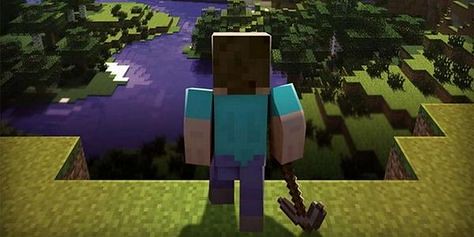This detailed image from the game Minecraft features the iconic blocky aesthetics that characterize the game. In the center stands the main character, Minecraft Steve, facing away from the viewer. He is easily identifiable with short, dark hair and a distinct outfit consisting of a short-sleeved aqua (or teal) shirt, dark blue (or purple) pants, and possibly dark brown boots. In his right hand, he holds a curved stone pickaxe with a gray head and a long, wooden handle, which is resting on the ground.

Steve is perched on an elevated piece of land, possibly a hill or mountain, overlooking an impressive, expansive scenery. This landscape includes a large body of deep blue water with reflections, surrounded by a mix of yellow-green and brown terrain, patches of shrubbery, and some trees. The waterway appears visually striking, sometimes interpreted as purple, and connects several islands or plots of land. Additionally, a small patch of snow can be spotted towards the center-left of the image, contrasting with the predominantly green landscape. The scene is rich and vibrant, capturing the game's blocky and textured world beautifully.